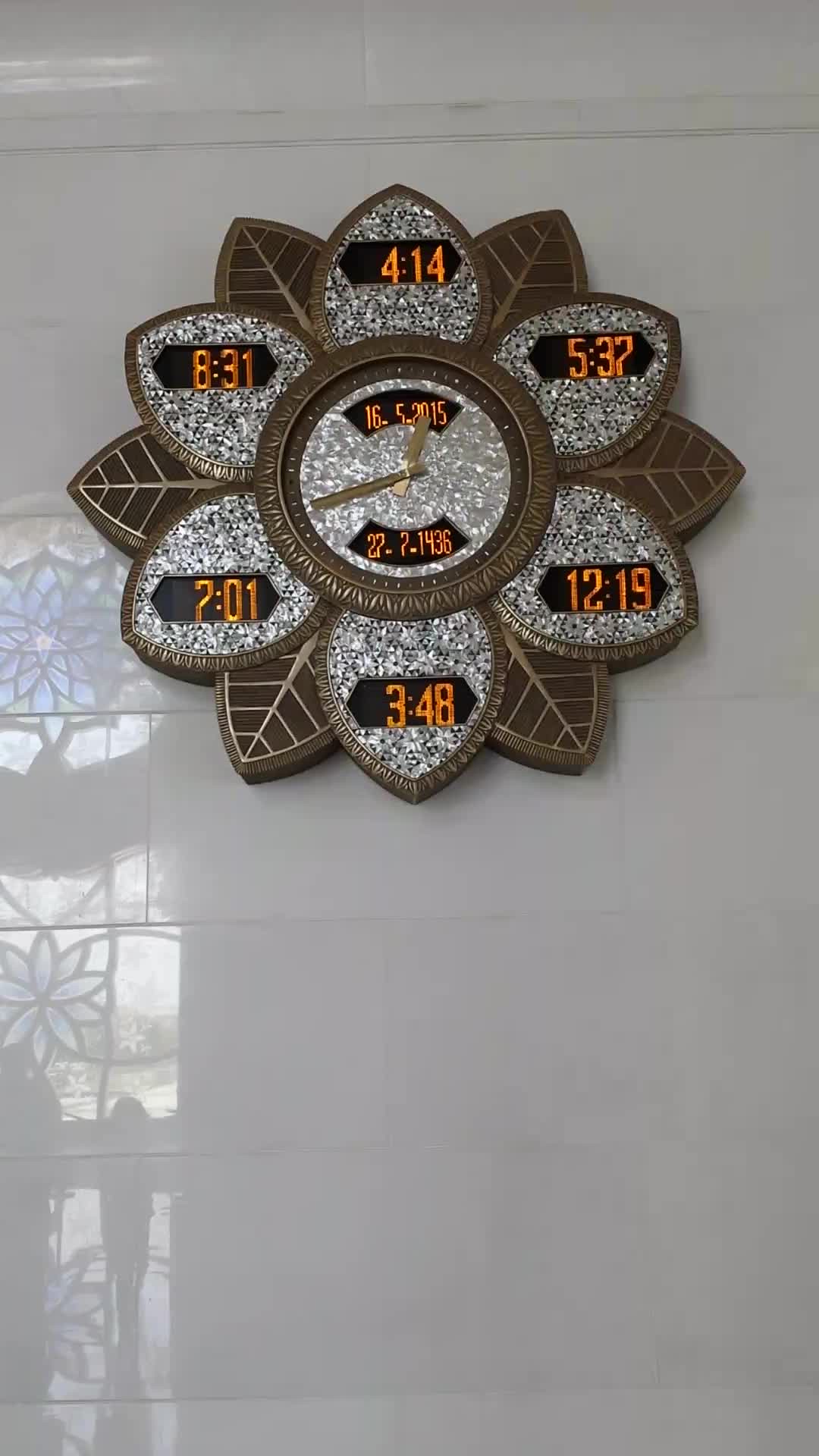The image, likely taken from a phone given its tall orientation, centers on an intricate clock designed to resemble a lotus flower. The clock's main petals and leaves exhibit a silver or granite finish, while the background leaves and the trim, as well as the concentric circles in the middle, display a brown wood grain texture. Each petal showcases different times, presumably representing various global locations. Positioned centrally towards the top of the clock is the date "16-5-2015," with another date, "27-7-1436," situated directly below it. The clock is mounted on a glossy, tiled laminate wall, which adds a reflective sheen to the image. In the bottom left corner, the reflection of a stained glass door or window adorned with various floral designs is visible, beyond which some greenery can be faintly seen.